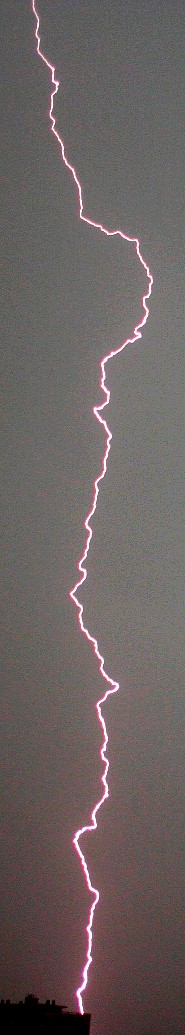This vertical photograph captures a dramatic lightning bolt against a grayish-violet sky, likely taken at nighttime. The bolt emerges from the top left of the frame, zigzagging downwards and occasionally jutting to the right, creating a labyrinth of pinkish-white light. It ultimately strikes a black structure, possibly a tree or building, located in the bottom left corner of the image. The striking contrast between the vivid lightning and the dark silhouette of the structure enhances the photo's intensity, making it a compelling snapshot of a thunderstorm. The monochromatic background sky further accentuates the brightness and dynamic path of the lightning bolt as it cuts through the heavens, filling the tall, thin frame with its electric energy.